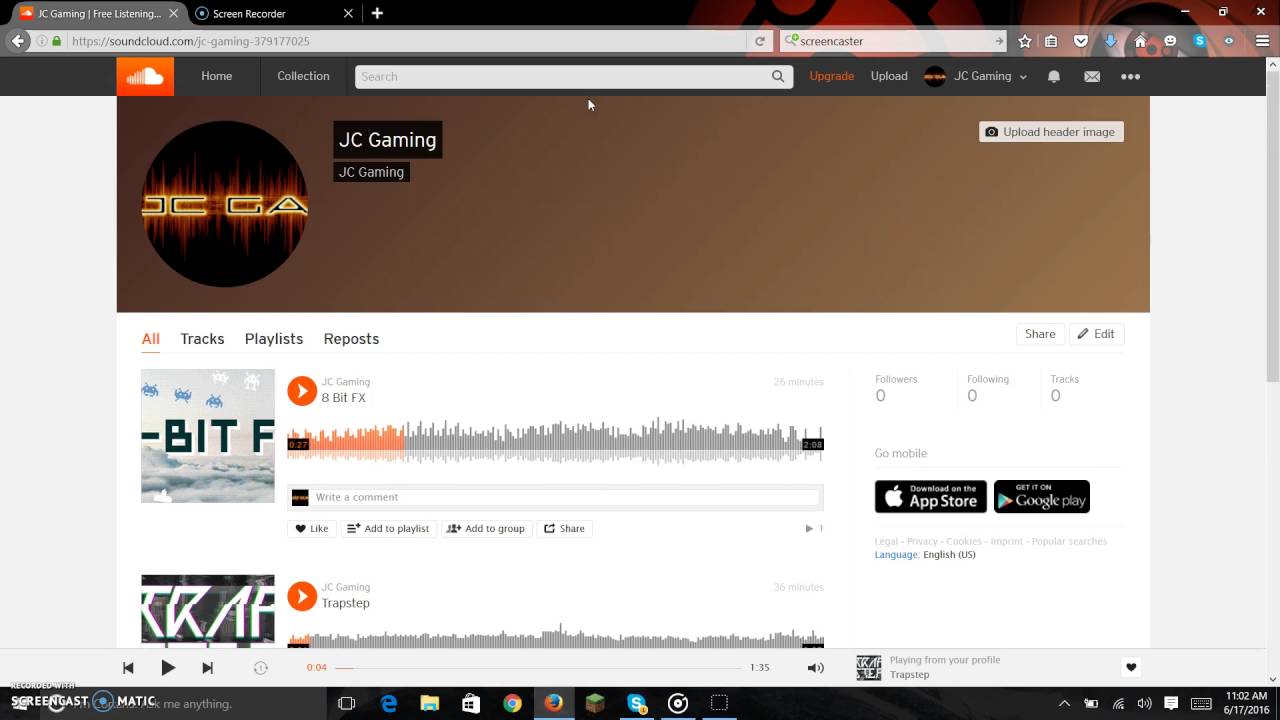**Detailed Caption:**

The image showcases the SoundCloud profile for a user named JCGaming. The profile features a distinctive logo—a black circle surrounded by vibrant, glowing flames. Within the circle, the initials 'JCGA' are emblazoned, with 'JC' representing JCGaming and 'GA' denoting Gaming. Below the captivating logo, there's text that reads "All Tracks Playlist Repost," accompanied by a display of the current track, which is titled "8-Bit FX" by JCGaming. Additionally, a sound meter bar is visible, indicating the audio levels of the track being played.

There is a comment section available under the track for listeners to share their thoughts. Another listed track titled "Trapstep" can be seen beneath the current one. The webpage indicates that SoundCloud is available for download via both the App Store and Google Play, with corresponding icons on the right side for users wishing to install the app.

It's worth noting that JCGaming currently has no followers, is following no one, and has no tracks listed on the profile. The image appears to be taken from a laptop screen, evident from the visible taskbar at the screen's bottom. The taskbar displays various icons, including E3, Explorer, file folders, a shopping icon, Microsoft Store, Google Chrome, Firefox, Minecraft, and Skype. The date and time are also visible in the bottom right corner of the screen. Overall, the caption provides a thorough look at JCGaming's SoundCloud profile and the available features for users wishing to engage with the platform via computer or mobile app.